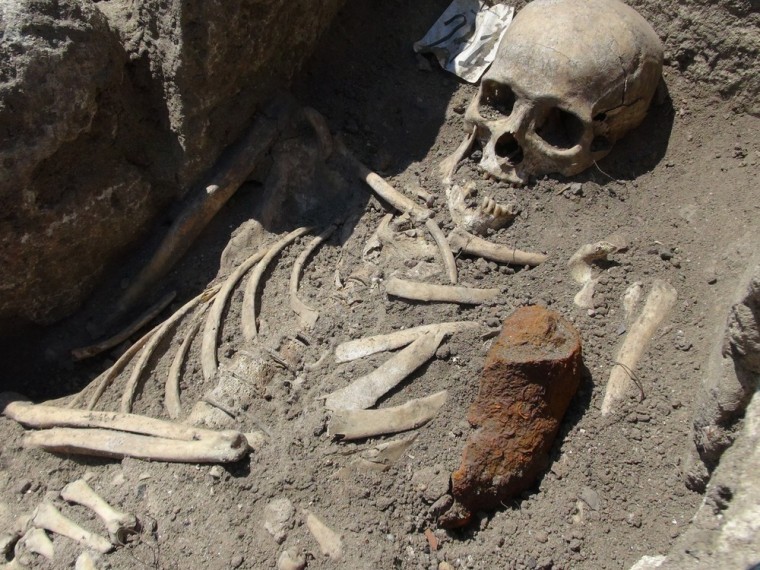The image depicts an uncovered grave revealing partially buried skeletal remains. The skull, positioned in the top right corner, has its mouth open and is partially covered in dirt. The rest of the skeleton is visible from the waist up, with prominent bones including the rib cage, spine vertebrae, and arms. Some bones are cracked and scattered, while parts are still buried. Adjacent to the ribs and the right arm, a brown-colored rock or object is noticeable. The ground consists of gray sand, and placed beside the skull is a white piece of paper with something written in black, though the text is indistinct. The grave appears to be surrounded by a rock wall, suggesting the skeleton is still within its original burial context.